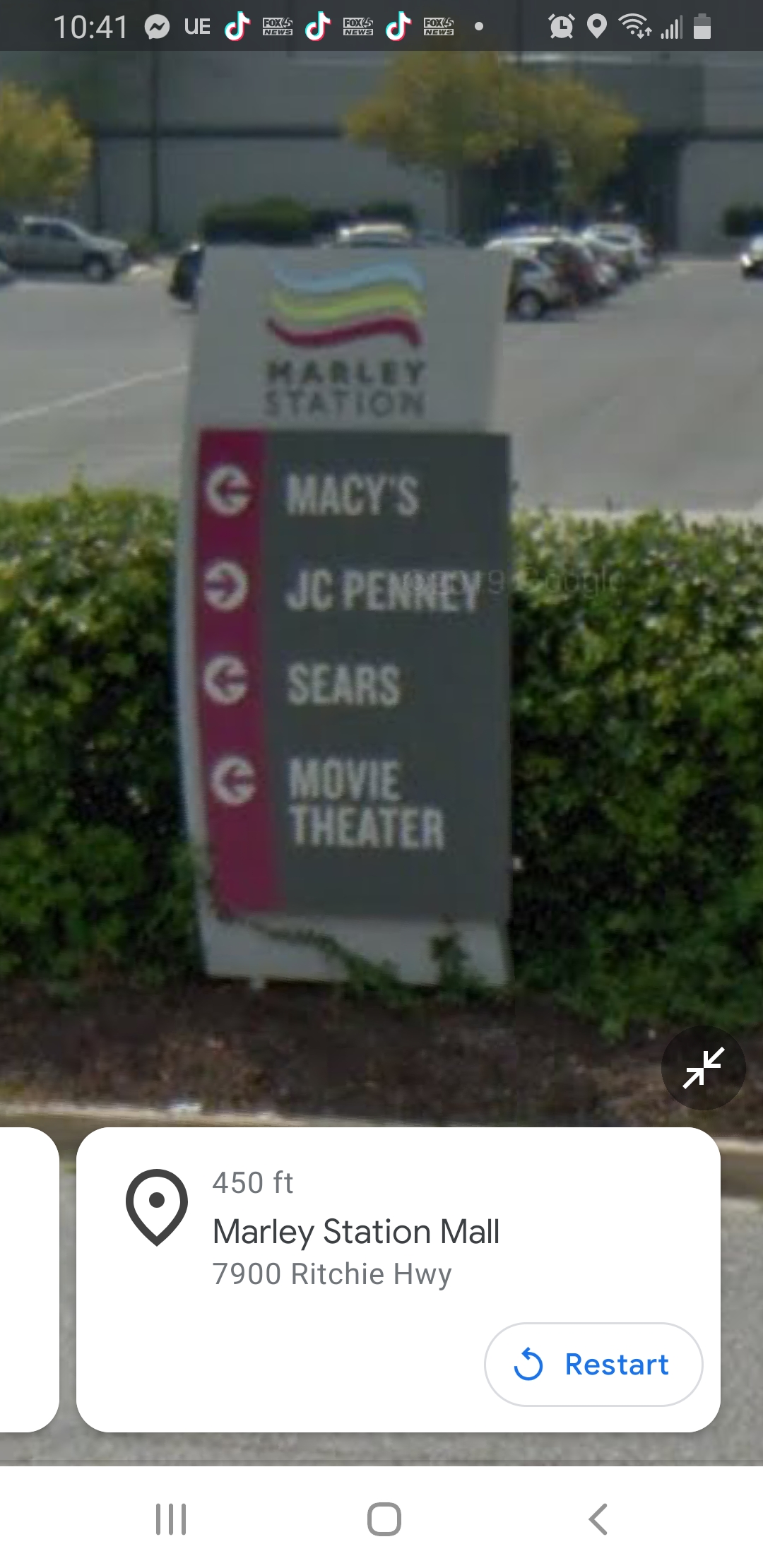The image is a screenshot from an Android phone displaying a Google Maps street view. The phone screen shows the time as 10:41, with active Wi-Fi, cellular data, and an alarm set. The battery is around 50%, and there are notifications from Facebook, TikTok, and other apps. The main focus is a street view of Marley Station Mall, located 450 feet away at 7900 Ritchie Highway.

In the image, a gray sign positioned in front of a green bush is prominent. The sign features three swirly lines in blue, green, and red, reminiscent of the Aquafresh logo, and reads "Marley Station." Below this is another section of the sign with directional arrows and store names: an arrow pointing left for Macy's, an arrow pointing right for JCPenney, an arrow pointing left for Sears, and another arrow pointing left for the movie theater. These arrows and labels are white on a gray background framed by a red border.

Behind the sign, there is a parking lot with various cars and some greenery, including trees and bushes, as well as a grayish building, likely part of the mall. The phone's screen also shows a white square at the bottom with a pinpoint marker and the text "450 feet, Marley Station Mall, 7900 Ritchie Highway." Additionally, there is a blue "Restart" button in the bottom right-hand corner and a black icon with two white arrows above it, presumably for resizing the image.